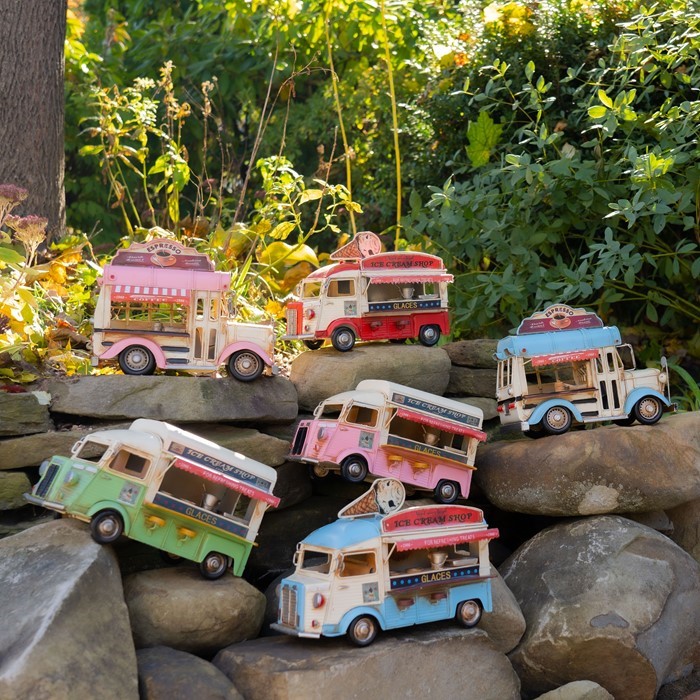The photo captures an outdoor scene showcasing a meticulously arranged collection of toy trucks on a pile of large, irregularly shaped rocks. Each toy truck resembles miniature versions of food vending vehicles, reminiscent of ice cream trucks or hot dog stands, adding a whimsical touch to the display. The trucks vary in vibrant colors: pink, red, blue, and green, with some featuring detailed designs of windows and service counters, as if they were genuine food trucks. Specific labels are visible on some trucks, with one prominently displaying "espresso" along with coffee graphics, and another labeled "ice cream shop" highlighted by images of ice cream cones. Two trucks are distinctly noted for not showing images but still bear the label "ice cream shop." Positioned artfully among the rocks, the trucks appear almost as though they might be navigating the rocky terrain. In the background, lush greenery including bushes, wildflowers, shrubs, and a significant tree trunk to the upper left, adds a naturalistic frame to this charming scene.